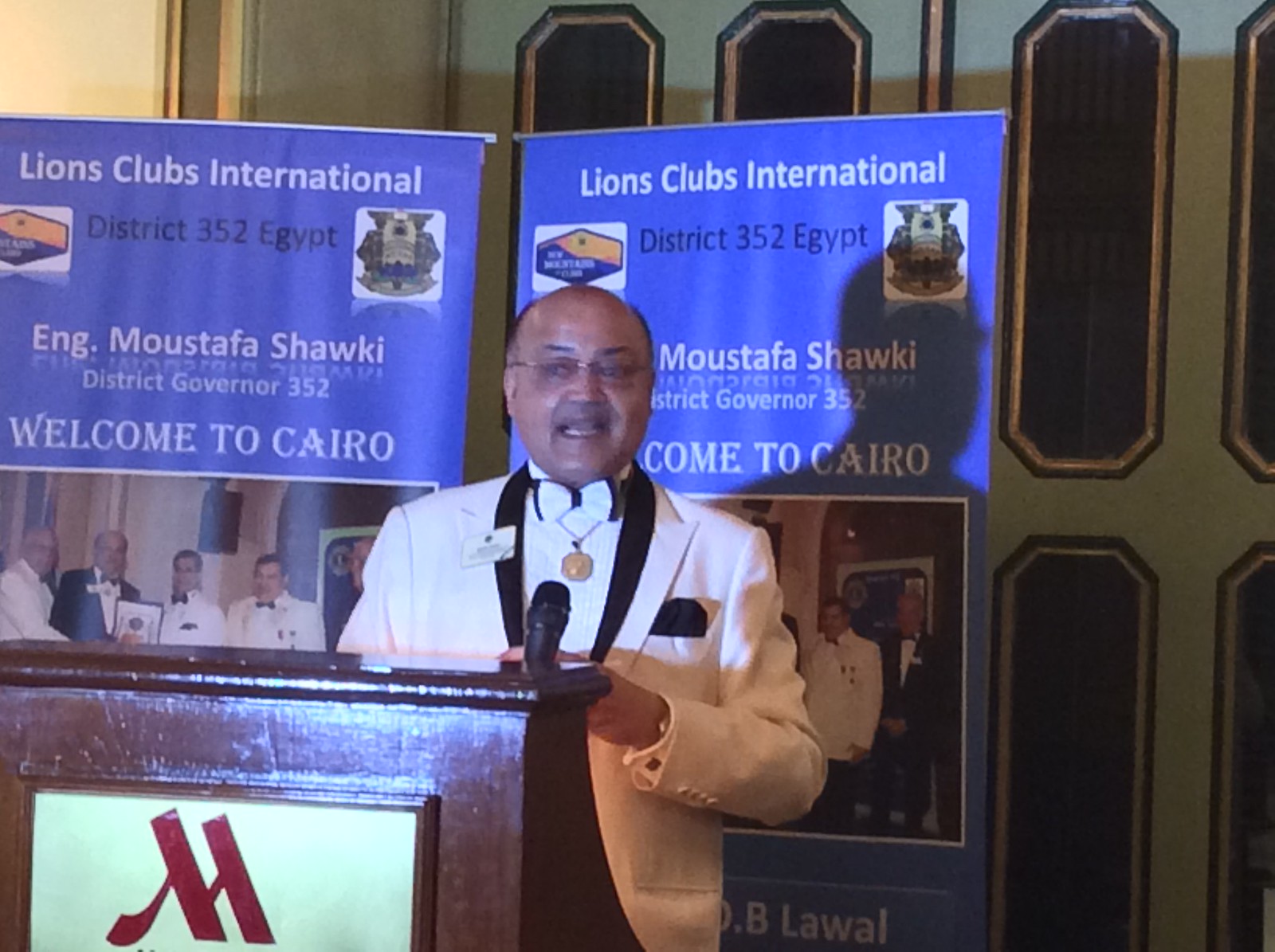The photograph captures a vibrant event at the Marriott Hotel in Cairo, hosted by Lions Club International, District 352, Egypt. Featured prominently in the image is an older, balding gentleman with glasses and a mustache, standing at a wooden lectern adorned with the Marriott's red stylized 'M' logo. He's dressed in a distinguished white tuxedo with black trim and a black and white bow tie. A gold medal hangs from a ribbon around his neck, just below his bow tie, accentuating his formal attire. A white card and a black handkerchief are neatly pinned to his lapel. The backdrop includes two large blue banners that repeat the inscription, “Lions Club International, District 352, Egypt,” and “Welcome to Cairo.” Each banner also features the name "Eng. Moustafa Shawki, District Governor, 532," alongside photographs of several men in suits. Despite the low lighting casting a prominent shadow on the background, the atmosphere of celebration and recognition is palpable, as the gentleman appears to be delivering a speech, possibly in acknowledgment of an award or a notable position within the organization. Behind him, a set of double doors with an intricate green, black, and gold design adds to the grandeur of the setting.